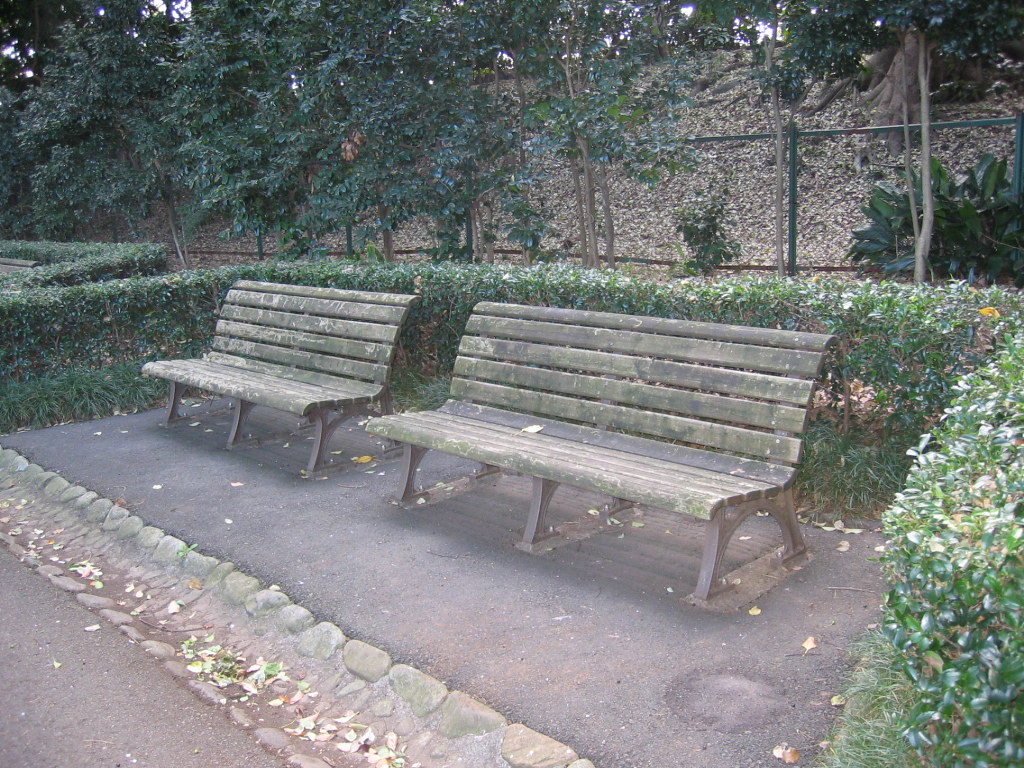The photograph captures a muted-color outdoor scene dominated by greens, grays, and browns. Two aged park benches, with greenish-gray, moldy, and possibly moss-covered wooden slats and metal legs, are positioned off a path within a small concrete alcove. The benches, each supported by three U-shaped metal frames, are surrounded by carefully trimmed green hedges that curve around them, forming a protective U-shape. The hedge is interspersed with speckles of lighter green and yellow. The ground beneath the benches is concrete with a distinctive grey circle in front of the bench on the right. Ahead of the benches, a line of stones creates a lip filled with dried leaves. Beyond the hedge, tall dark green trees rise, and a chain-link fence stands in front of a hill covered in additional trees, bushes, and mulch. At the very top of the image, a sliver of white sky is visible.